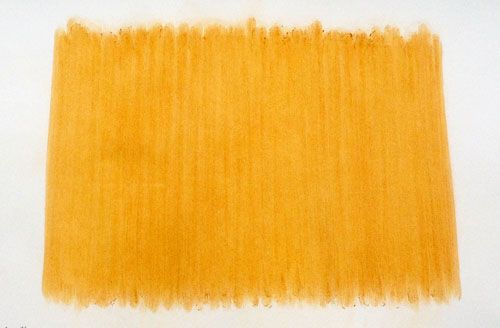The image depicts a drawing on an off-white canvas or paper, featuring a block of tall, vertical brushstrokes in a burnt yellow or golden orange hue. The strokes stretch almost from the top to the bottom of the page, beginning about half an inch to an inch in from either side, and are centered uniformly between the four edges of the canvas. The brushstrokes create a patternless, repetitive texture resembling the color of hay or wheat, with no additional elements such as text, signatures, or background details. Near the top, there are darker specks of debris, likely residues from the crayon or pastel medium used to create the strokes.